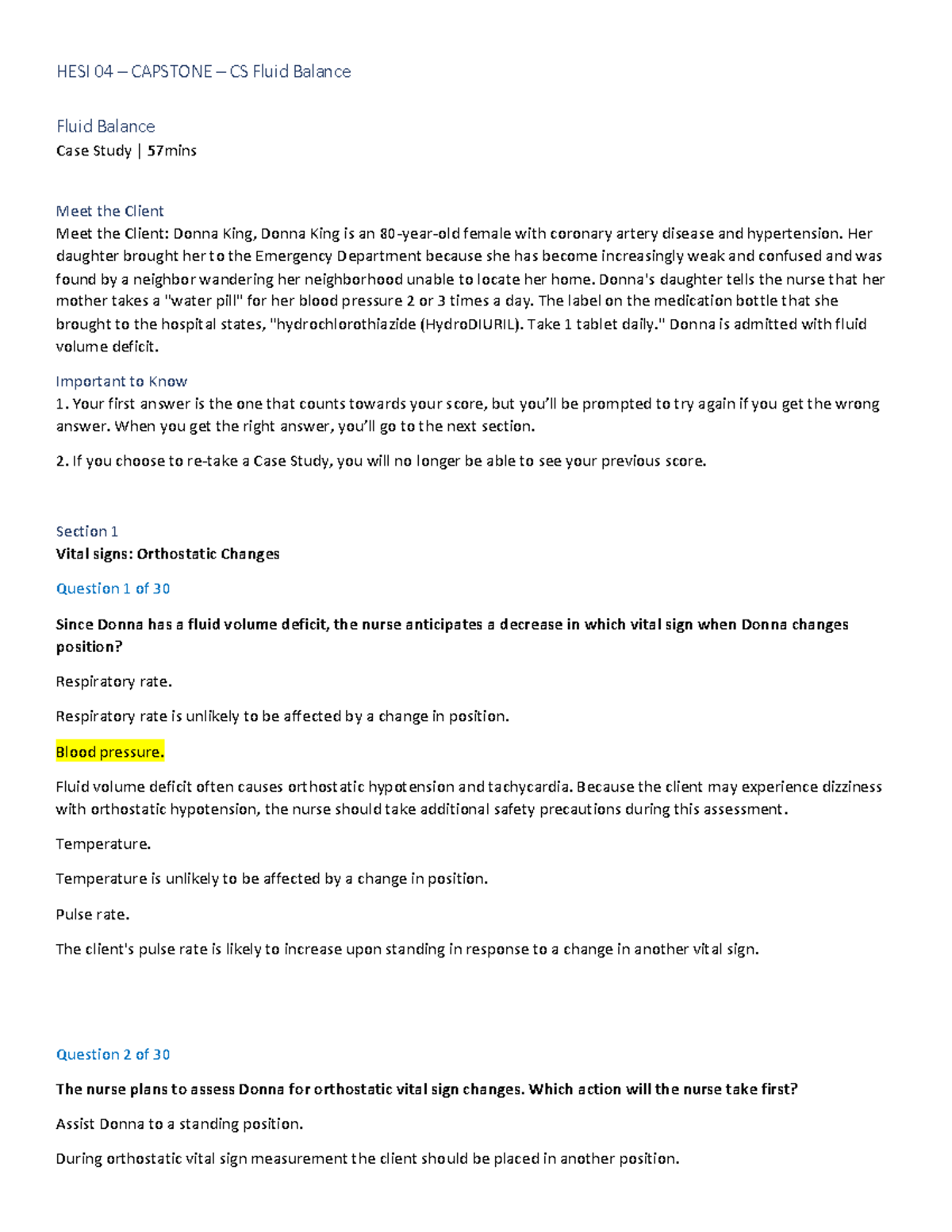The image contains a detailed case study document titled, "Fluid Balance," displayed in a formal or article-like structure. At the top, in blue text, is the section heading "Meet the Client." 

Following this, there is a paragraph in a darker font that provides information about the client: "Meet the Client: Donna King. Donna King is an 80-year-old female with coronary artery disease and hypertension. Her daughter brought her to the emergency department because she has become increasingly weak and confused and was found by a neighbor wandering her neighborhood, unable to locate her home. Donna's daughter tells the nurse that her mother takes 'the water pill' for her blood pressure two or three times a day. The label on the medication bottle that she brought to the hospital states hydrochlorothiazide, take three tablets daily. Donna is admitted with fluid volume deficit."

Below this detailed client introduction, there is a section titled "Important to Know," which is subdivided into two parts:
1. Vital signs, orthostatic changes.
2. Questions one through 30, with a specific focus on blood pressure highlighted in yellow, followed by a list of five different considerations related to blood pressure management and monitoring.

Additionally, the image notes that the overall case study duration is 57 minutes.